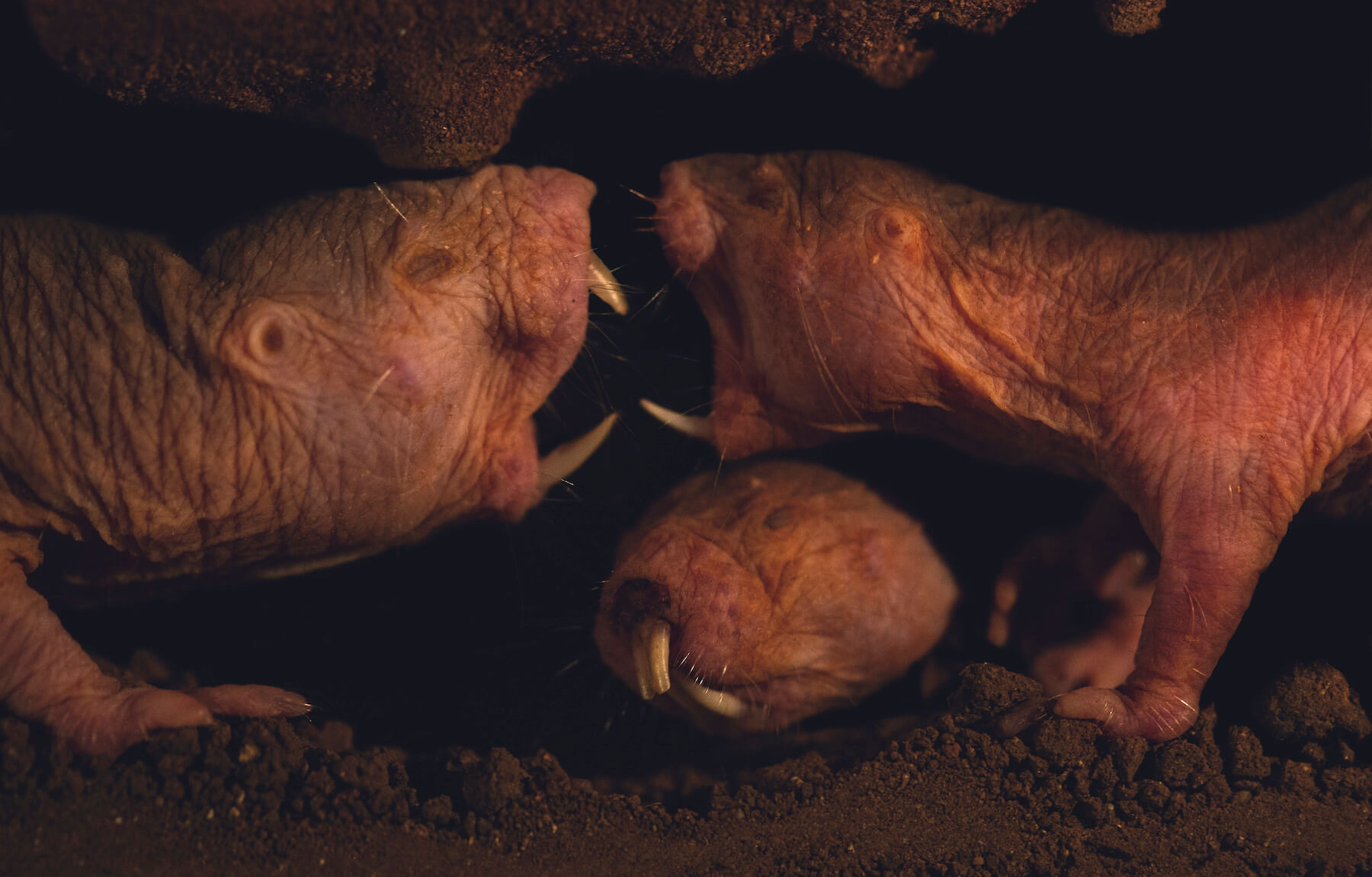This photograph captures a scene from within a mole rat den, likely situated underground. The top and bottom edges of the image are framed by clumps of brown dirt, creating the illusion of a subterranean environment. The central background is shrouded in darkness, accentuating the stark contrast of the three prominently featured hairless, pinkish-brown mole rats.

Two of these peculiar creatures are facing each other, their wrinkled, leathery skin illuminated in the dim light. Each has its mouth wide open, baring long, sharp teeth—one sporting a prominent fang from the top jaw and another from the bottom, while the other has a single, menacing tooth pointing upwards. Their small, round ears and single visible eyes add intensity to their almost confrontational posture, suggesting a form of communication or dispute. Their robust front legs are visible, emphasizing the heavy build of these unusual rodents.

Beneath these two, nestled in the middle of the frame, lies the head of a third mole rat. This one faces forward with its mouth closed, yet the distinct, prong-like teeth remain noticeable. It appears somewhat passive in contrast to the energetic interaction above it. The overall ambience of the photograph is mysterious and slightly foreboding, a stark depiction of life in the underworld of these enigmatic creatures.